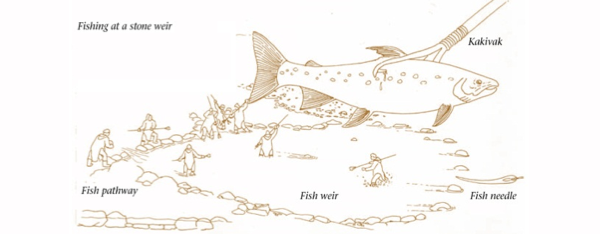The image is a detailed sketch with a horizontal rectangular shape and a white background, showcasing various methods of fishing at a stone weir. At the top left corner, the diagram is labeled "Fishing at a Stone Weir" in black text. The central feature is a large fish skewered by a traditional three-pronged wooden spear, labeled "kakivak," illustrated in brown and situated in the top right portion of the image. Below the fish, an oval-shaped layout of small stones represents a pond, with labeled areas: "Fish Pathway" on the left, "Fish Weir" at the center, and "Fish Needle" on the right, all indicated in blue text. Inside and around this pond, various figures, depicted in orange outline, are actively engaged in fishing using the spear-like tools, appearing to stab or aim at the fish. The detailed sketch captures the communal and traditional fishing methods employed around the stone weir, emphasizing the collaborative nature of the activity.